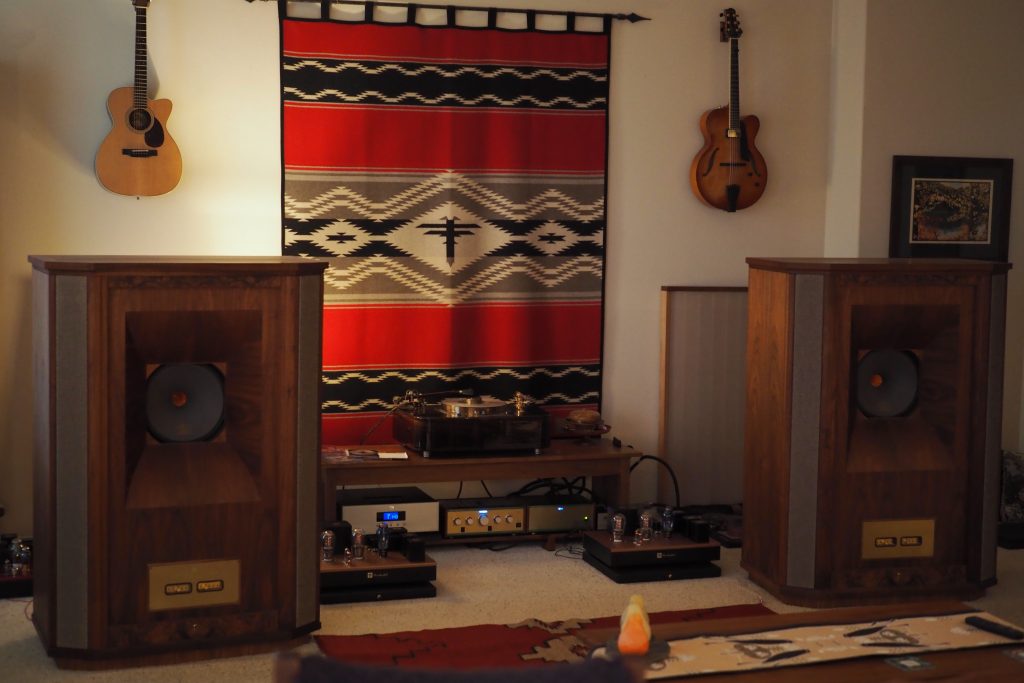This photograph captures a cozy, vintage music room in someone's house, likely designated for a passionate music lover. The room is viewed in landscape orientation and features prominently a richly colored tapestry against the back wall with red, black, gray, and white stripes, possibly of a Navajo or Southwestern design. Flanking the tapestry, two guitars are elegantly hung on either side, contributing to the musical décor.

Central to the composition is a low table or shelf holding an electronic record player, surrounded by various receivers and stereo equipment adorned with numerous dials and lights, indicative of a finely tuned sound system. On the floor, slightly right of center, sits a pink Himalayan salt lamp, adding warmth to the ambiance.

Commanding attention on the left and right sides of the room are two tall, vintage wooden speakers with gold panels at their base, likely from the 70s, complementing the overall retro aesthetic. The ground features a matching Navajo-styled rug, tying the room’s thematic elements together seamlessly. This detailed assemblage vividly reflects the personality and preferences of its music-enthusiast owner.